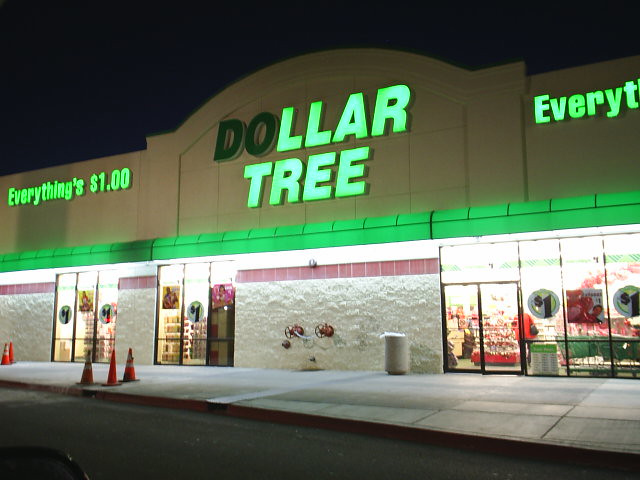A photograph of the exterior of a Dollar Tree store, captured at night, prominently features the store's illuminated sign across the top. However, the "DO" in "DOLLAR" is unlit, resulting in only "LLAR TREE" being visible on the left side of the sign. The store's slogan, "Everything's a Dollar," appears on the right, partially obscured, showing only "every" and "T." The entrance consists of two double glass doors, flanked on the right by glass panes divided into three sections, with additional window segments on either side. A solid middle section of wall between these windows houses two red fire hose spigots protruding outward. Three orange traffic cones are positioned on the left side of the sidewalk, near the edge where the sidewalk meets the street.